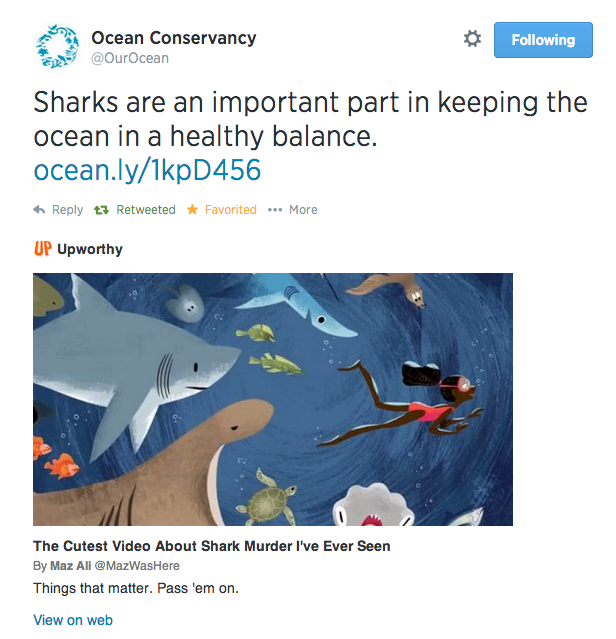The image is a screen capture from a social media site, featuring a post by Ocean Conservancy on their "Our Ocean" campaign. At the top, there's a teal and blue circular icon adorned with illustrations of sea creatures, including dolphins and sharks. Beside the icon is a gray cogwheel. A blue button with white text labeled "Following" is prominently displayed below the header.

The main post text, in black, reads: "Sharks are an important part of keeping the ocean in a healthy balance." Below this, a blue hyperlink is provided: "ocean.ly/1KPD456." Interactive options are listed in gray, including "Reply," "Retweeted," and "Favorited." The gray text also mentions "Morn" followed by three dots, and "Upworthy".

The image accompanying the post is illustration-style, set against a navy background. In it, various marine animals are depicted: a whale, a green sea turtle, a gray shark, a white jellyfish, and some green fish. An African American woman with black hair, dressed in a pink bathing suit, is swimming among them. Surrounding her are bubbles and orange clownfish.

Below the illustration, there's a caption: "The cutest video about shark murder I've ever seen" by Maze Alley (@mazewashere). It concludes with, "Things that matter, pass them on," and a blue "View on web" link at the bottom. The image quality is excellent, capturing even the smallest details, including a goofy-looking gray shark with googly eyes at the bottom of the illustration.